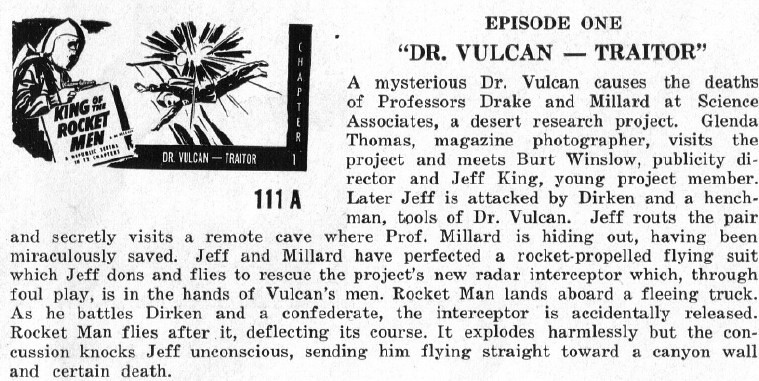This detailed caption describes a vintage black-and-white illustration likely from a comic book or radio program from the 1930s or 1940s. The image on the upper left features a man in a space suit wielding a ray gun, indicative of a futuristic superhero theme. The text adjacent to the image reads "King of the Rocket Men," with the title "Dr. Vulcan Traitor" prominently displayed. The content seems to be an excerpt from either a magazine or a promotional piece for "Episode 1: Dr. Vulcan Traitor." The narrative introduces the sinister Dr. Vulcan, who orchestrates the deaths of Professors Drake and Millard at Science Associates, a desert research project. Glenda Thomas, a magazine photographer, visits the project and meets Burt Winslow, the publicity director, along with Jeff King, a young project member. Jeff is later ambushed by Durkin and an accomplice, who are operatives of Dr. Vulcan. After fending off the attackers, Jeff secretly visits a cave where Professor Millard, miraculously saved, is hiding. Together, they have perfected a rocket-propelled flying suit. Jeff dons the suit to intercept a radar device hijacked by Vulcan's men. In an action-packed sequence, Rocket Man boards a fleeing truck, battles Durkin and a Confederate, and deflects the device's course, but the ensuing explosion renders him unconscious, sending him hurtling towards a canyon wall and imminent death.